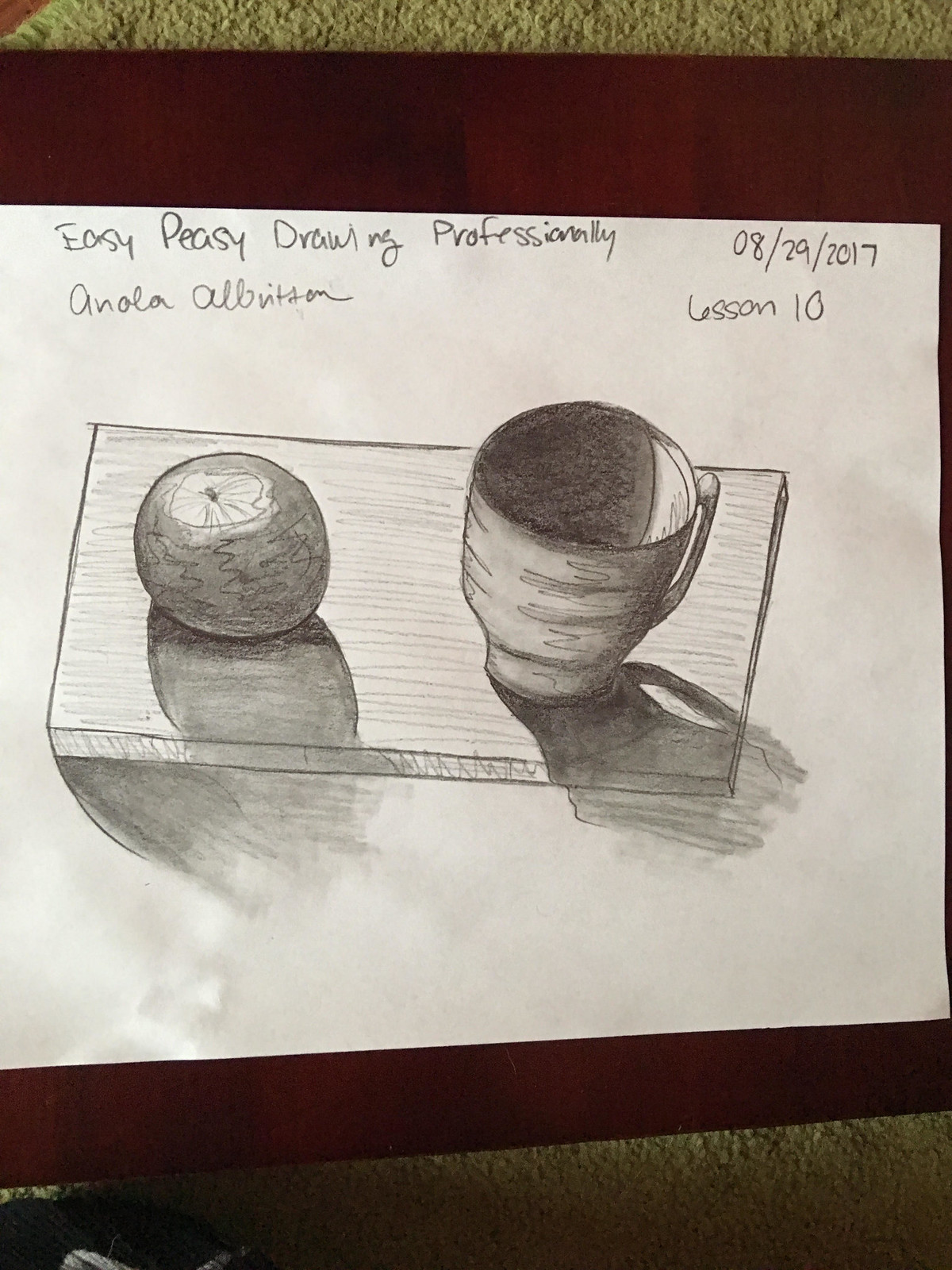The image showcases a detailed pencil sketch of a mug and an orange resting on a piece of wood, drawn on a horizontal sheet of white paper. The sketch is rendered in black and white. Above the drawing, handwritten text reads "Easy Peasy Drawing Professionally." Directly below that, the name "Enola Albertson" is inscribed, followed by the date "08 29 2017" and the notation "Lesson 10." The white paper bearing the sketch lies on a thick-surfaced burgundy-colored table, beneath which a beige shag carpet is visible. In the far left-hand corner of the composition, part of a person's foot donned in a navy blue yarn slipper with white trim can be seen.